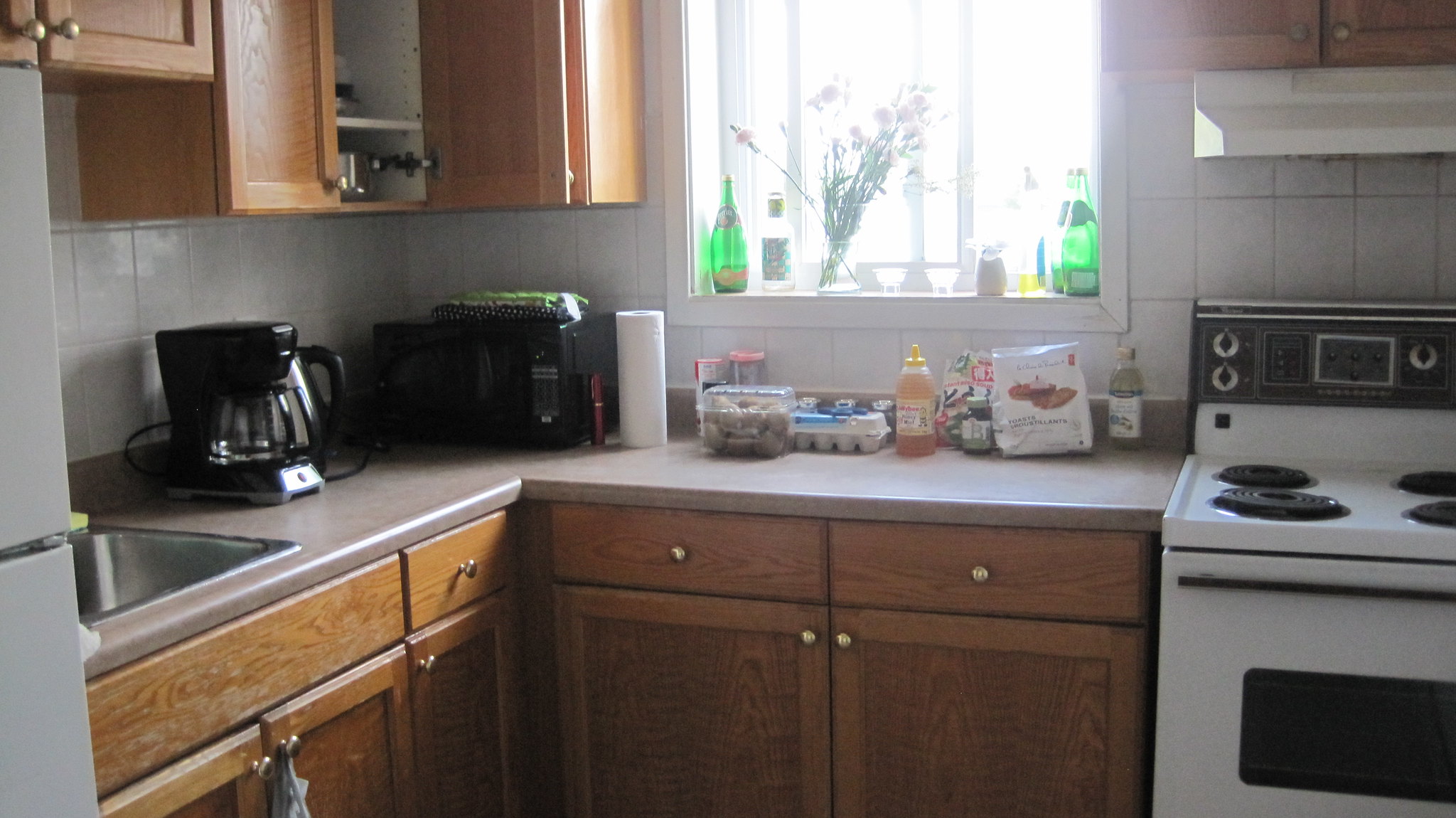This detailed image captures a cozy kitchen scene, starting from the bottom left corner with the edge of a refrigerator curving up toward the top. Adjacent to the fridge is a glimpse of a light brown shelf with a gold handle. Moving right, there's a quarter-view of a shelf with a knob in its bottom right corner, followed by a longer shelf, roughly twice the length, also with a knob in the bottom right corner. The door next to this shelf is open, revealing a single white shelf inside.

To the immediate right is a brightly-lit window, framed in white trim that extends halfway down the image. The window sill hosts a charming arrangement: a green bottle on the left, a clear bottle beside it, some reaching flowers, and another green bottle in the corner. Beneath the window, extending under the shelves, is a wall that continues toward and above the stove area.

Centered below the wall is a white stove with a black control panel featuring three silver knobs. The stove's front is white, while the handle stretching across it is black. To the right of the stove, a countertop extends back towards the refrigerator, where a silver sink can be partially seen. Above the sink area, a black coffee pot is positioned with a microwave overhead, leading right to a series of various items including bags, an egg carton, and paper towels.

Below these objects are two rectangular drawers with center knobs, followed by two larger cabinets. The cabinet door on the left has a knob in the top left corner, while the one on the right has a knob in the top right corner. To the immediate right of the stove is a compact wooden surface with a small drawer above and an equally small door beneath it. This rich description encapsulates the entire kitchen, giving a vivid sense of its layout and contents.